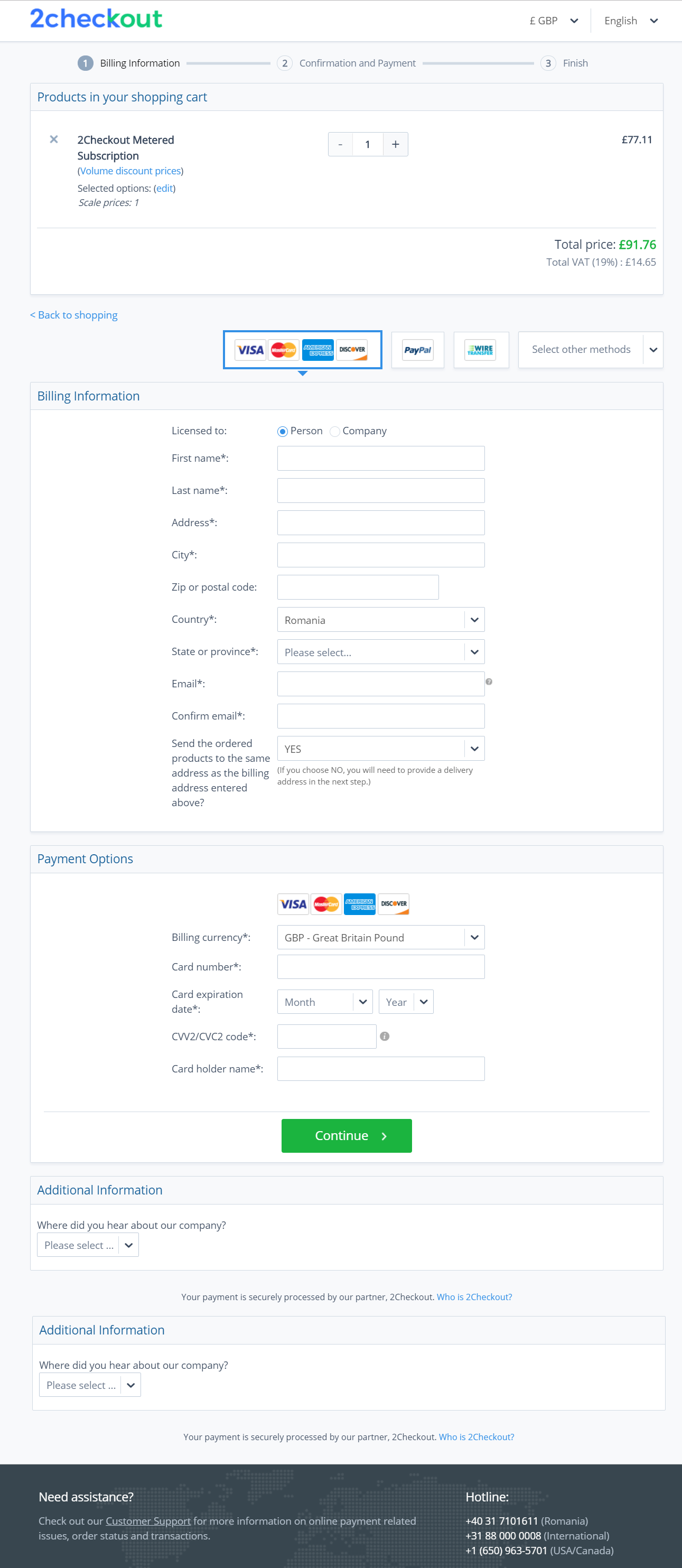A rectangular screenshot shows the checkout screen of a subscription-based app. The background is light gray with a detailed footer at the bottom, featuring a light gray background adorned with square shapes forming a globe, highlighting the Northern Hemisphere. The footer contains white text stating: "Need assistance? Check out our customer support for more information on online payment related issues, order status and transactions, hotline, plus 4031-710-1611, Romania, plus 3188-000-0008, International, plus 1-650-963-5701."

At the top of the main body of the page is a blue-titled box that reads, "Products in your shopping cart." Inside this box, the following text is displayed: "To checkout meter subscription, Volume discount prices, Selected options, Scale prices, 1." The item listed has a price of £77.11. Below this information is the total price for the subscription.